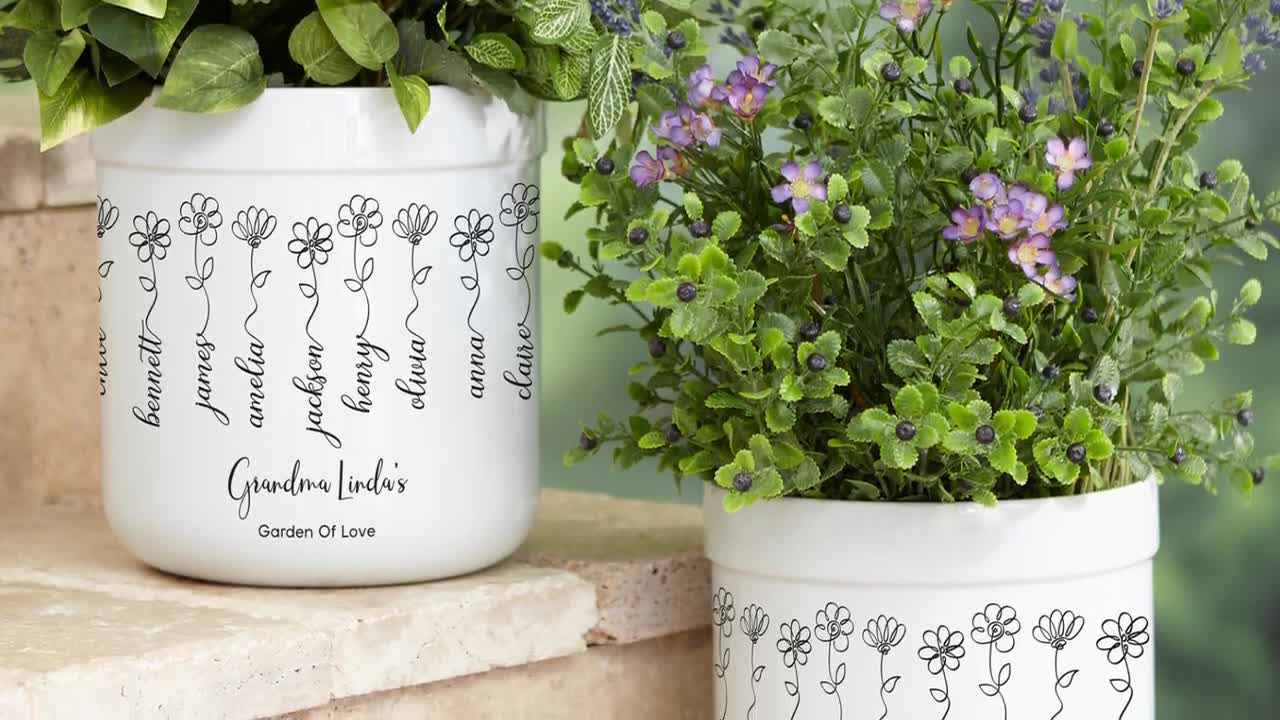This close-up photograph showcases two white ceramic planters, adorned with thin, hand-drawn doodles of simple daisies. These flowers are intricately designed, with the names Bennett, James, Amelia, Jackson, Henry, Olivia, Anna, and Claire written in cursive along their stems, seamlessly blending into the floral motif. The planters are labeled "Grandma Linda's Garden of Love," suggesting a personalized touch for displaying the names of loved ones. The planters are placed on marble steps, with one pot positioned on a lower step and the other on an upper step. The greenery within the pots appears generic and potentially artificial, with one plant featuring small purple blossoms. The background of the image is slightly blurred, displaying some greenery that seems photoshopped, emphasizing the focus on the detailed and heartfelt design of the planters.